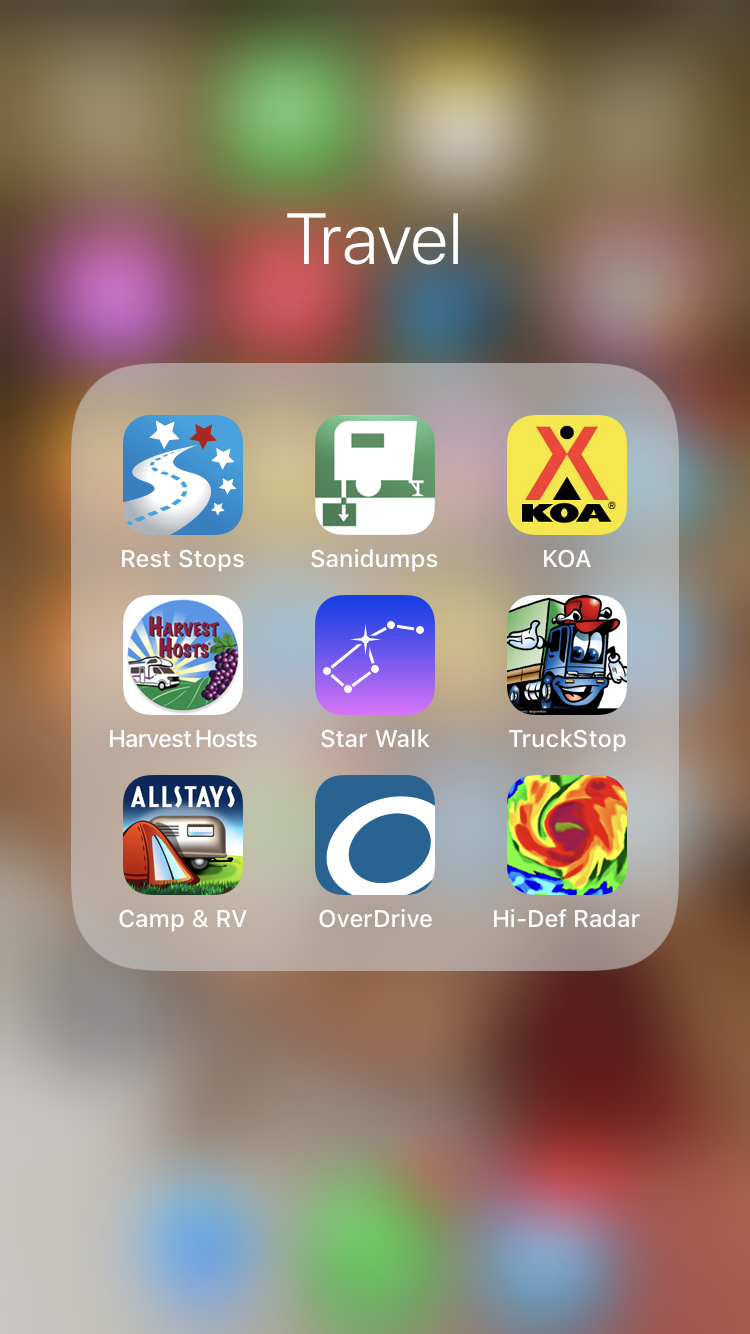This is a detailed screenshot taken from a phone displaying a collection of travel-related applications. Centered at the top of the screen is the word "Travel" in white text. Below it is a neatly organized grid of small application icons, arranged in a three-by-three layout within a square with rounded corners.

On the top row, from left to right:
1. Rest Stops
2. Sani Dumps
3. KOA (Kampgrounds of America)

In the middle row, from left to right:
1. Harvest Hosts
2. Truck Stops
3. KOA

On the last row, from left to right:
1. Camp & RV
2. OverDrive
3. HiDef Radar

Each app icon is a small, rounded square that represents the brand of the respective app. For instance, the icon for Starwalk resembles a white constellation in the shape of a kite, set against a gradient background that transitions from blue at the top to pink at the bottom. The OverDrive icon features a simple "O" set against a blue backdrop. This organized collection of apps under the category "Travel" provides users with a variety of resources for planning and navigating their journeys.